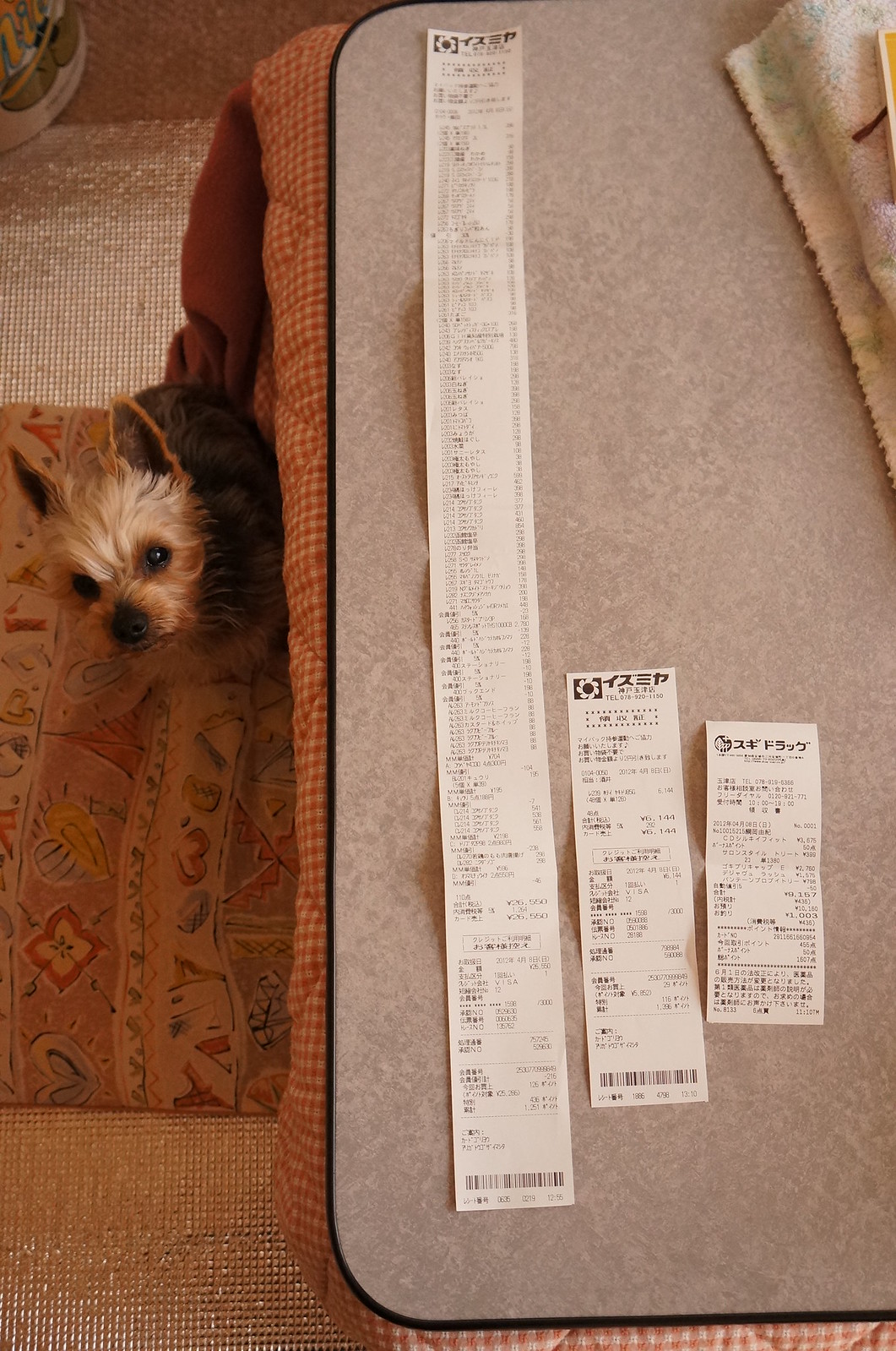A vertical photograph taken inside a cozy home captures an intriguing scene. On the right side of the image, there is a piece of furniture which could be a bed, a couch, or an ottoman. Spread out on this furniture are three receipts, each with Japanese text. The receipt on the far left is exceptionally long, possibly one of the longest receipts ever seen. To its right, a comparatively smaller receipt is placed, followed by an even smaller receipt on the far right. Adding an adorable touch to the scene, a small dog peeks out from underneath the furniture on the left side of the image, its curious face emerging just slightly.